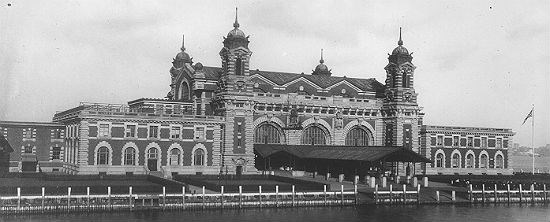The image depicts an old black-and-white photograph of a large, castle-like building that spans the entire width of the horizontal frame. The sky is filled with gray clouds, contributing to the overcast and somber mood of the scene. The building itself is substantial in size, constructed from brick with arched windows and dark gray rooftops adorned with spikes at the sides. Manicured lawns and bushes are visible in the foreground, indicating well-maintained landscaping. There's also a road running along the bottom edge of the photograph. This grand structure gives an impression of housing royalty or serving as a significant government edifice. Additionally, a United States flag can be seen flying, suggesting a notable American landmark, possibly Ellis Island, with its distinct large steeples and architectural style. The setting captures a moment in history, frozen in a monochromatic palette of black, white, and numerous shades of gray.